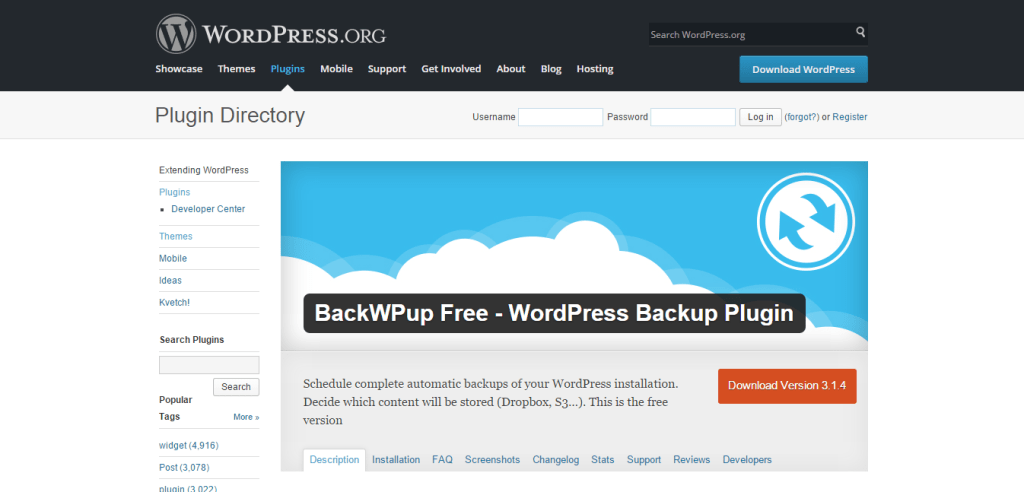The image depicts the WordPress.org website interface. On the right-hand side, there is a search bar that allows users to search for specific articles. Below the WordPress.org header, there's a navigation menu featuring buttons such as Showcase, Themes, Plugins, Mobile, Support, Get Involved, About, Blog, and Hosting. The 'Plugins' section is currently selected and highlighted in blue.

Users can also log in via a section that includes fields for the username and password, with options to register if they haven't already, or to recover a forgotten password. 

Below this, there's a featured plugin titled "BackWPup – Free WordPress Backup Plugin" showcasing two blue circular arrows indicating backup activity. The background features blue skies with fluffy white clouds. 

A gray box beneath the title contains a brief description: “Schedule complete automatic backups of your WordPress installation. Decide which content will be stored. Dropbox, S3 – this is the free version.” The 'Description' tab is selected, offering further details.

Additional tabs available include Installation, FAQ, Screenshots, Changelog, Stats, Support, Reviews, and Developers. There is also a download button for version 3.1.4 highlighted in red.

On the left side of the screen, there are more expandable sections like Plugins, Developer Center, Themes, Mobile, Ideas, and Popular Tags, which offer various widgets and posts related to WordPress plugin development and themes.